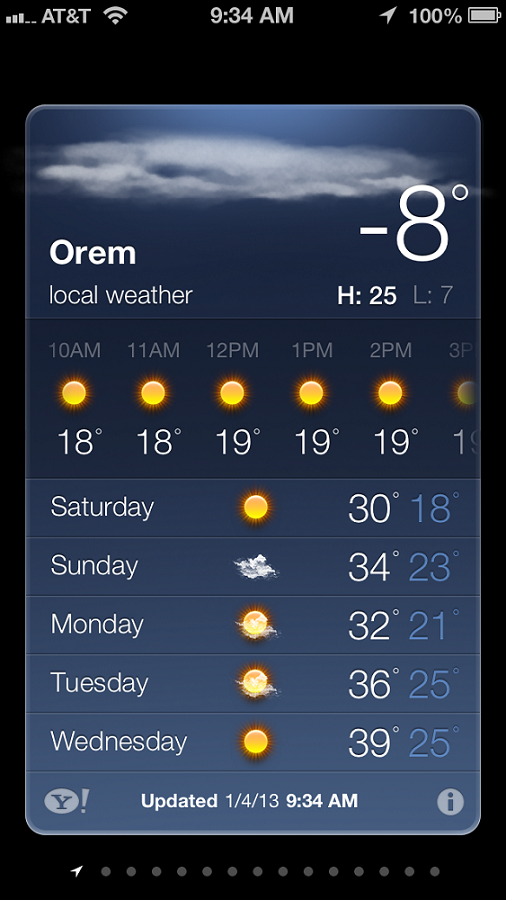This image is a smartphone screenshot with a predominantly black background. At the top, the status bar displays several elements: on the far left, there is the network bar accompanied by the label "AT&T" and a Wi-Fi signal icon. Centered in the top bar is the current time, "9:34 AM," while the top-right corner shows the location services icon, a 100% battery charge indicator, and a full battery icon, all in white.

Below the status bar, there is a weather application pop-up featuring a blue background with cloud imagery. The weather app shows the current location as "Orem" and provides the local weather conditions, indicating an unusually frigid temperature of -80 degrees. 

The forecast includes a timeline from "10 AM to 2 PM," predicting sunny weather with temperatures ranging from 18 to 19 degrees. The app also displays a weekly forecast covering Friday through Wednesday, with temperatures and weather icons (sunny, partly cloudy, cloudy) representing daily conditions.

Text within the weather application is primarily white, offering clear readability against the blue and black backgrounds. Weather icons add visual aids, such as a yellow sun for sunny conditions, enhancing the informative nature of the display. The time and date of the last update are also noted, ensuring the viewer that the information is current.